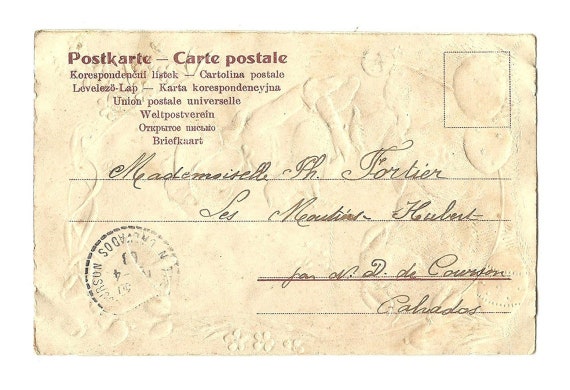This horizontally aligned, rectangular postcard features an intricate, albeit faded, design on a light tan or beige background. The edges appear somewhat rough and worn, indicative of its age. At the upper left, printed in brown, are multiple variations of the word "postcard" in different languages: "Postkarte," "Carte postale," and "Postale" in red. Below these, lines of cursive writing in black ink are present, though the exact words are difficult to decipher. The addressed side of the postcard includes phrases like "Mademoiselle PH Fortier" and "Hubert," suggesting it might be French, despite the unclear readability of other words. A circular postal stamp appears in the lower left corner, and while faint, it adds to the postcard's authenticity and vintage feel. The upper right corner features a small, empty square where a postage stamp would typically be placed. The postcard's overall tone is accentuated by subtle hints of light yellow and pink, adding to its charming antiquity.